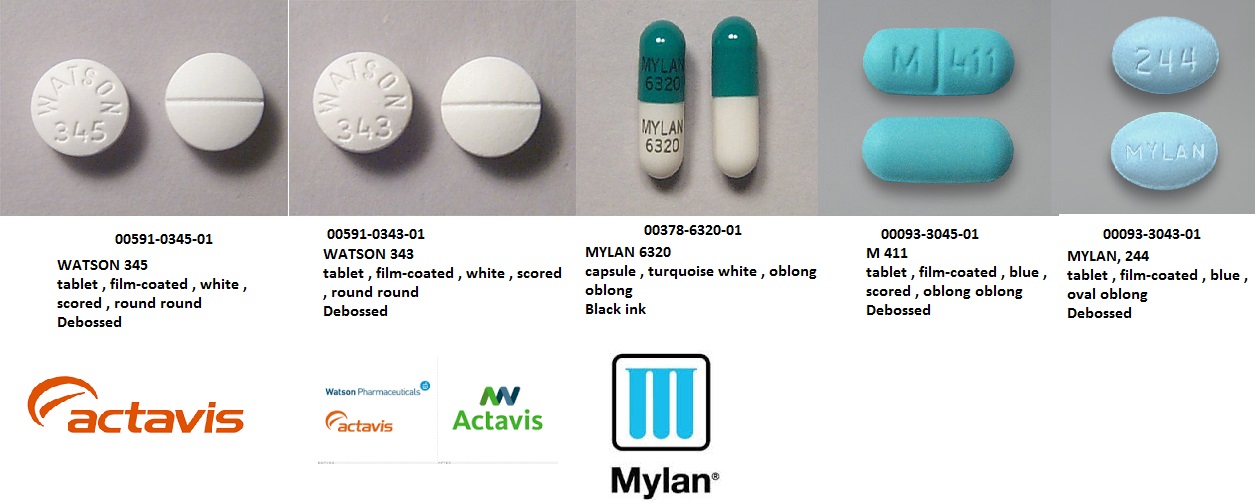The image consists of five separate photographs, each displaying two different sides of various medications. 

1. **First Image**: On the left, a pill with text engraved on the top side, and on the right, its reverse side devoid of any markings. 

2. **Second Image**: Similar to the first, it features a medication with a text-engraved top side on the left, and a plain reverse side on the right.

3. **Third Image**: Following the same pattern as the first two images, the pill on the left displays engraved text on the top side, with the plain reverse side shown on the right.

4. **Fourth Image**: The pill on the left has a top side displaying letters and numbers, while its reverse side is not shown. 

5. **Fifth Image**: Both pills in this image have engraved text on both sides. The left one is labeled "244," and the right one is labeled "MYLAN."

Beneath these images, there are descriptive labels including numbers and brand names: "Watson 345," "Watson 343," "Mylan 6320," "M411," and "Mylan 244," listed respectively from left to right. Additional information is provided, detailing the type of tablet or capsule (e.g., film-coated), the color, scoring, and shape (e.g., round or oblong), as well as the brand names.